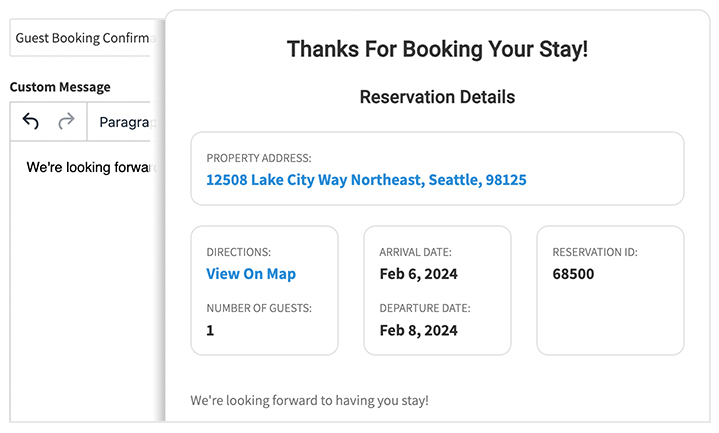This is an image showing a confirmation page from a website, verifying a booking. The header of the page reads, "Thanks for booking your stay," with a title in the center labeled "Reservation Details." Below the title, there is a prominent box displaying the property address: 12508 Lake City Way, NE Seattle, WA 98125. Within this box, there are three smaller centered boxes.

The first box contains a hyperlink labeled "Directions," allowing users to view directions on a map. Under this link, it mentions "Number of guests: 1." The second box provides the booking dates: "Arrival date: February 6, 2024," and "Departure date: February 8, 2024." The third box includes the "Reservation ID: 68500."

Underneath these details, the page reassures with the message, "We're looking forward to your stay." This confirmation appears as a pop-up, partly obscuring the underlying content. Visible parts of the underlying content include a message stating "Guest booking confirmed" and a segment labeled "Custom message." There are arrows pointing left and right, and part of the text with the word "Paragraph" is also visible but cut off.

The website's design is primarily in black and white, with the exception of two blue hyperlinks, adding a touch of color to the otherwise monochromatic layout.